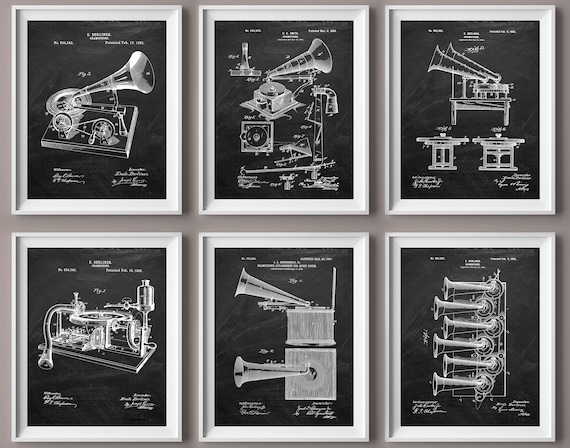This image showcases six framed prints, arranged neatly in two rows of three. The white wooden frames with a black matte border give a cohesive look to the black and white drawings. These highly detailed sketches resemble patent illustrations of various phonographs or record players, each highlighting different parts and inner workings of the devices. The backgrounds of the images are black, creating a chalkboard-like effect, and the white chalk-style drawings are accompanied by small, intricate labels and descriptions, though the text is too small to decipher. The top left image displays a complete, functional phonograph, while the center top image details various parts and their connections. The top right image and others in the bottom row further explore multiple phonograph assemblies and different components, including various horns.